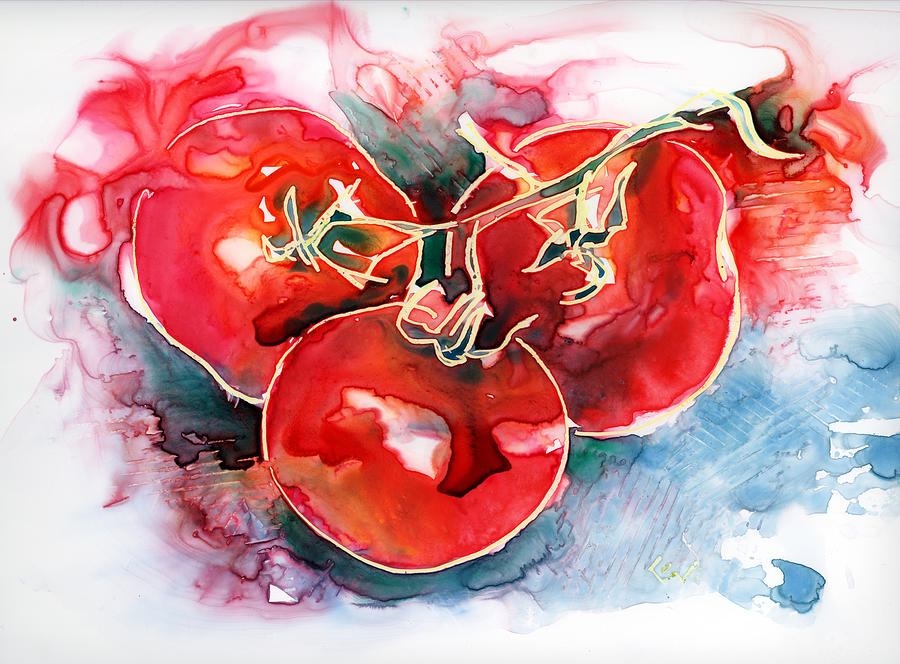This image vividly captures a watercolor painting of three bright red tomatoes attached to a green vine. The tomatoes dangle in the foreground with no visible support, bringing a sense of natural suspension. The background is primarily white, enhancing the tomatoes' rich red color. Surrounding the tomatoes are delicate watercolor patterns, including a splash of blue in the bottom right corner, subtle red watermarks, and hints of green interspersed throughout the image. At the top of the tomatoes, watermarks in green and pink add a touch of artistic flair, making the composition feel both dynamic and tranquil.